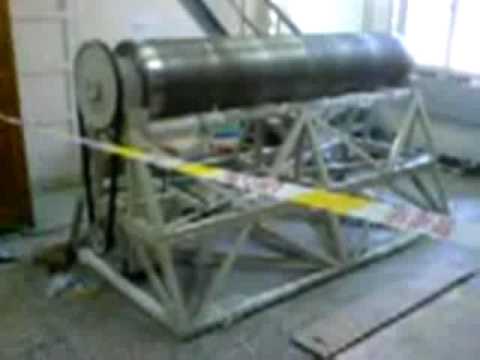A horizontally positioned, long cylinder with shades of silver, dark gray, and light gray is displayed on a metal rack resembling sawhorses. The cylinder, with a flat circular end on the left, appears to be part of a larger piece of machinery. The structure is supported by a silver metal base composed of various rods and cut-out components. Beneath the equipment, the concrete floor is marked with yellow and white outline tape, potentially indicating a restricted access area. In the background, a set of windows allows bright daylight to flood into the room, casting light over the entire scene. The machinery is situated near a stairwell, identifiable by the slanting wall on its right. The overall image is blurry, adding a level of ambiguity to the exact details of the machinery.